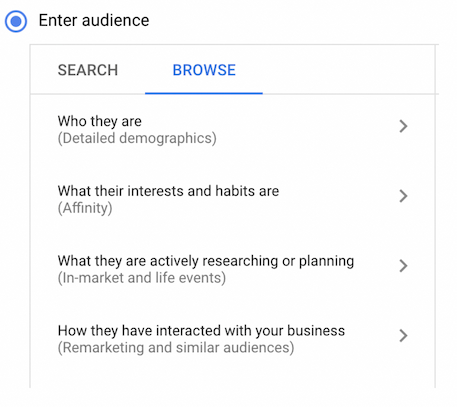This screen capture appears to be from a website or application interface, specifically a section dedicated to audience segmentation. At the upper left corner, there is a blue radio button labeled "Enter Audience." Directly beneath this header, there is a segmented box with two categories: "Search" in gray text and "Browse" in blue text, indicating that the "Browse" category is currently selected.

Below these categories is a line divider, under which four options are listed:

1. **Who They Are**: Displayed in black text, with "Detailed Demographics" noted in parentheses. A right arrow icon is located next to this option.
2. **What Their Interests and Habits Are**: Indicated with "Affinity" in parentheses alongside arrow icons.
3. **What They Are Actively Researching or Planning**: This category includes "In-market and Life Events" in parentheses.
4. **How They Have Interacted with Your Business**: Featuring "Remarketing and Similar Audiences" in parentheses.

These elements suggest a detailed audience targeting or segmentation tool designed to help users categorize and understand their audience based on various criteria.